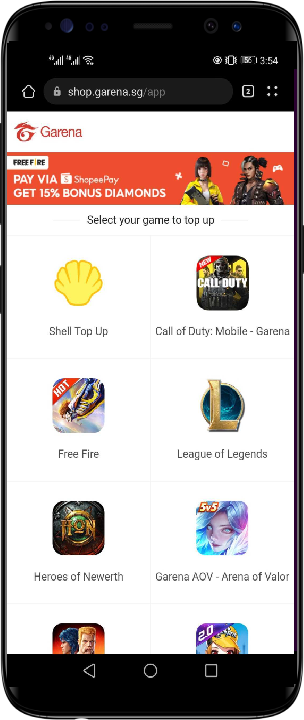The image features a mobile phone displaying a webpage from Garena, a well-known gaming platform. At the top of the page, the prominent Garena logo is visible, characterized by a stylized "G" adorned with flame or cloud-like design. Just beneath the logo is a striking banner with a promotional offer that reads, "Pay via ShopEatPay, get 50% bonus diamonds." Adjacent to this banner is a smaller tag labeled "Free Fire."

The webpage layout includes vivid, computer-generated images of two game characters, suggesting playable avatars within the Garena platform. Following this visual appeal, a subtitle prompts users with, "Select your game to top up."

In a grid-like arrangement, several game icons accompanied by their titles are arrayed below the prompt, showcasing eight different games. Starting from the top left, the games are listed as follows:
1. Shell Top Up
2. Call of Duty Mobile Garena
3. Free Fire
4. League of Legends
5. Heroes of Newerth
6. Garena AOV - Arena of Valor

The remaining two icons are partially visible, displaying only half of their visual representations, with their game titles cropped out of the view within the user interface of the mobile webpage.